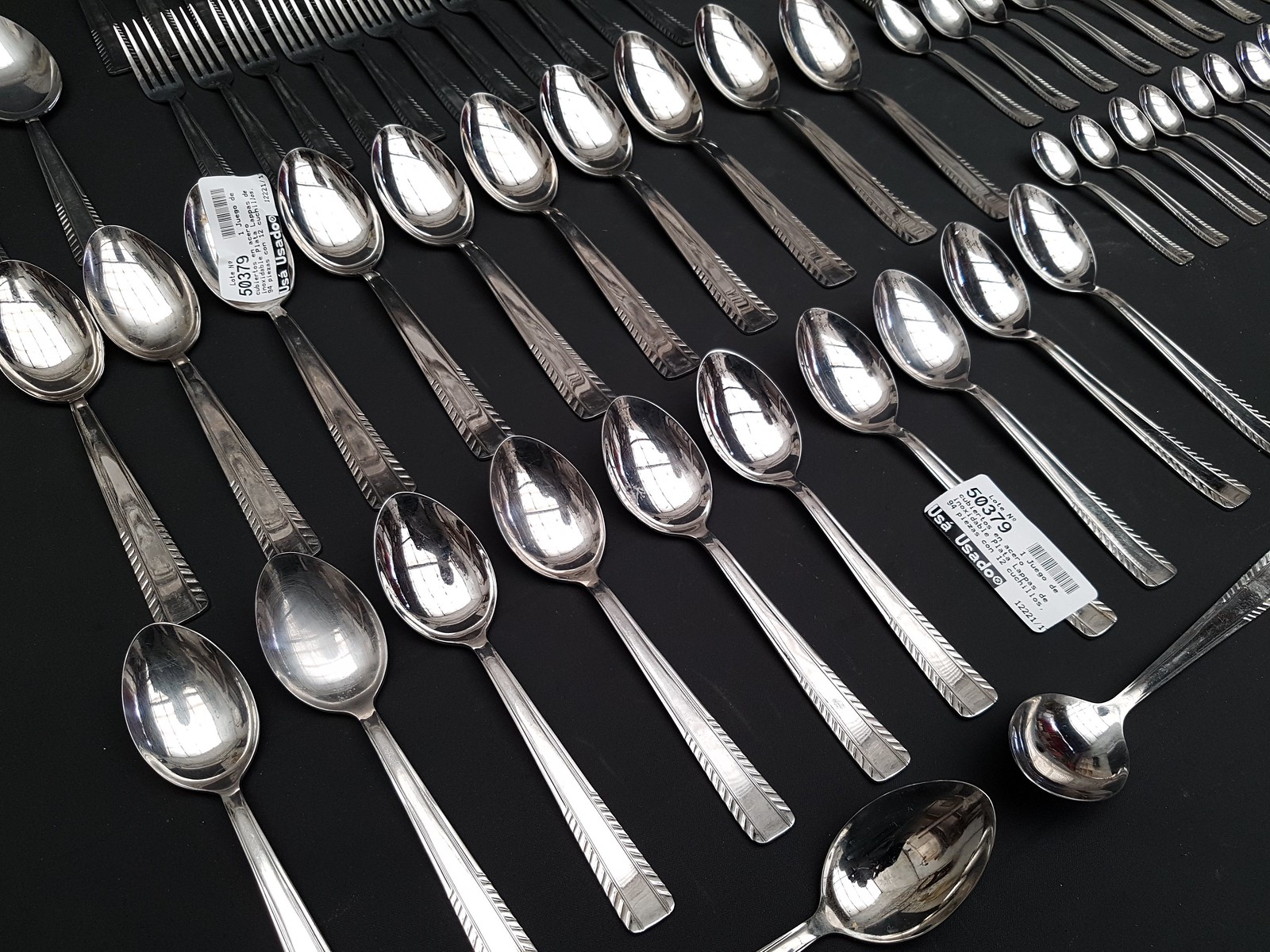The photograph captures an overhead view of a meticulously arranged assortment of mainly spoons and some forks laid out on a medium dark gray to black fabric surface. The cutlery appears to be either plain metal or potentially silver, though the quality is indeterminate. All pieces are meticulously organized by size and shape, creating a uniform pattern with matching designs. Two rows of spoons are prominently displayed, gradually decreasing in size from left to right and angling towards the top left corner of the frame. The top right corner features a row of five smaller spoons, likely teaspoons for espresso or coffee. The forks are concentrated in the middle upper part of the image. Two of the spoons are tagged with white stickers containing barcodes and the text “USA Usado 50379,” suggesting they are second-hand and possibly for sale. The overall impression is of a well-curated display of used cutlery, possibly in a store setting.